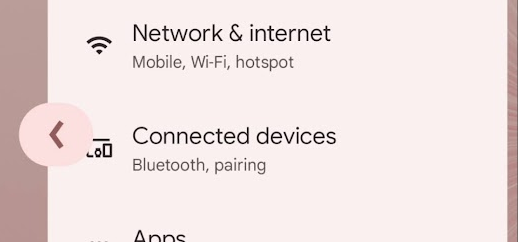The image depicts a smartphone menu screen, primarily featuring the "Network and Internet" settings. The background utilizes a gradient of brown taupe with subtle red hues, transitioning to the rightmost 10% which carries the same base color dotted with light gray striations. In the center-left portion, an oval button is prominent, colored in a dark brick brown and emblazoned with a back arrow icon.

At the top of the menu, bold black text reads "Network and Internet," followed by subheadings "Mobile, Wi-Fi, Hotspot." An icon on the left side, showing a full Wi-Fi connection with all three bars highlighted, accompanies this section. Further down, the text "Connected Devices, Bluetooth, Pairing" is listed, alongside an icon depicting a laptop with accompanying phone and watch symbols. The bottom portion of the menu is slightly truncated but reveals the word "Apps."